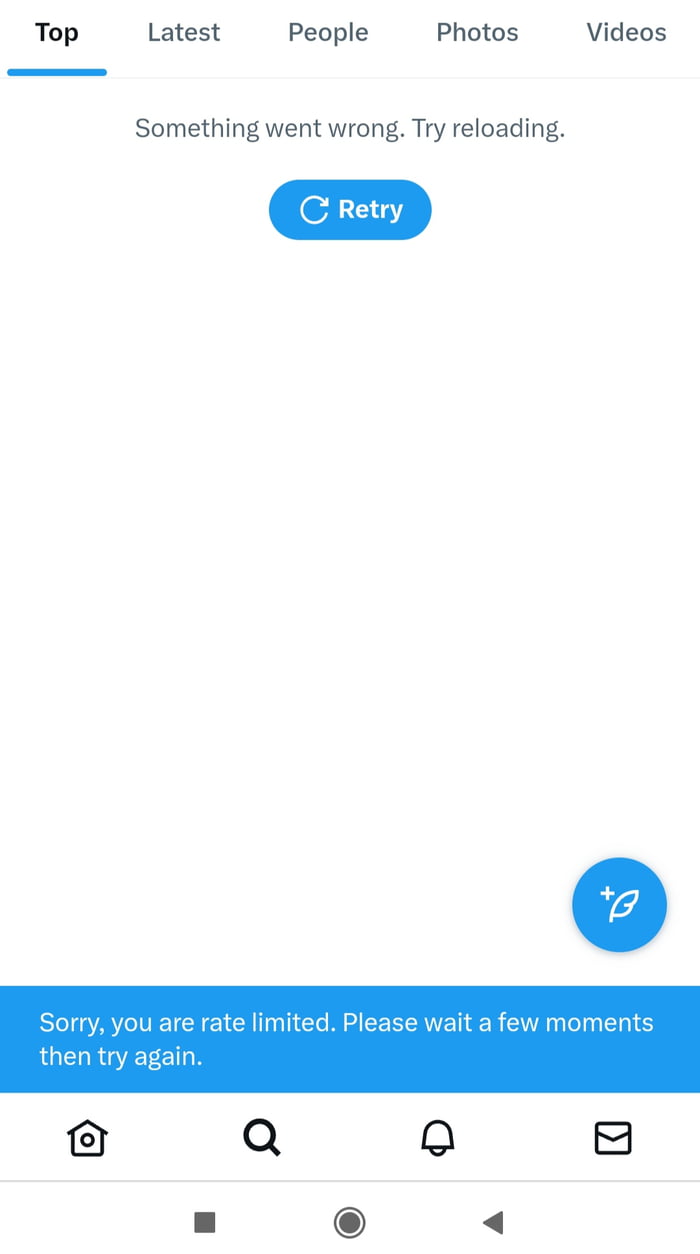The image seems to be a screenshot from a mobile app on a smartphone. At the top of the screen, there is a navigation bar with tabs labeled "Top," "Latest," "People," "Photos," and "Videos." The "Top" tab is currently selected, which is indicated by a blue underline and black text, while the other tabs are grayed out.

In the center of the screen, a message displays, "Something went wrong. Try reloading." Beneath this message is an orange button featuring a reload icon that forms an infinity loop with an arrow, and the button is labeled "Retry."

At the bottom of the screen, there is a navigation bar that includes icons for Home, Search, Notifications, and Email. Just above this navigation bar, there is a blue banner with white text that reads, "Sorry, you are rate limited. Please take a few moments, then try again." Above this banner is a blue circle icon with a feather and a plus sign inside it.

Additionally, there appears to be music controls at the very bottom, including a square stop button, a circle with a dark dot representing the record button, and a sideways triangle play button, suggesting playback controls for audio.

Overall, the screen indicates a rate limit error in the app, prompting the user to reload or try again later.